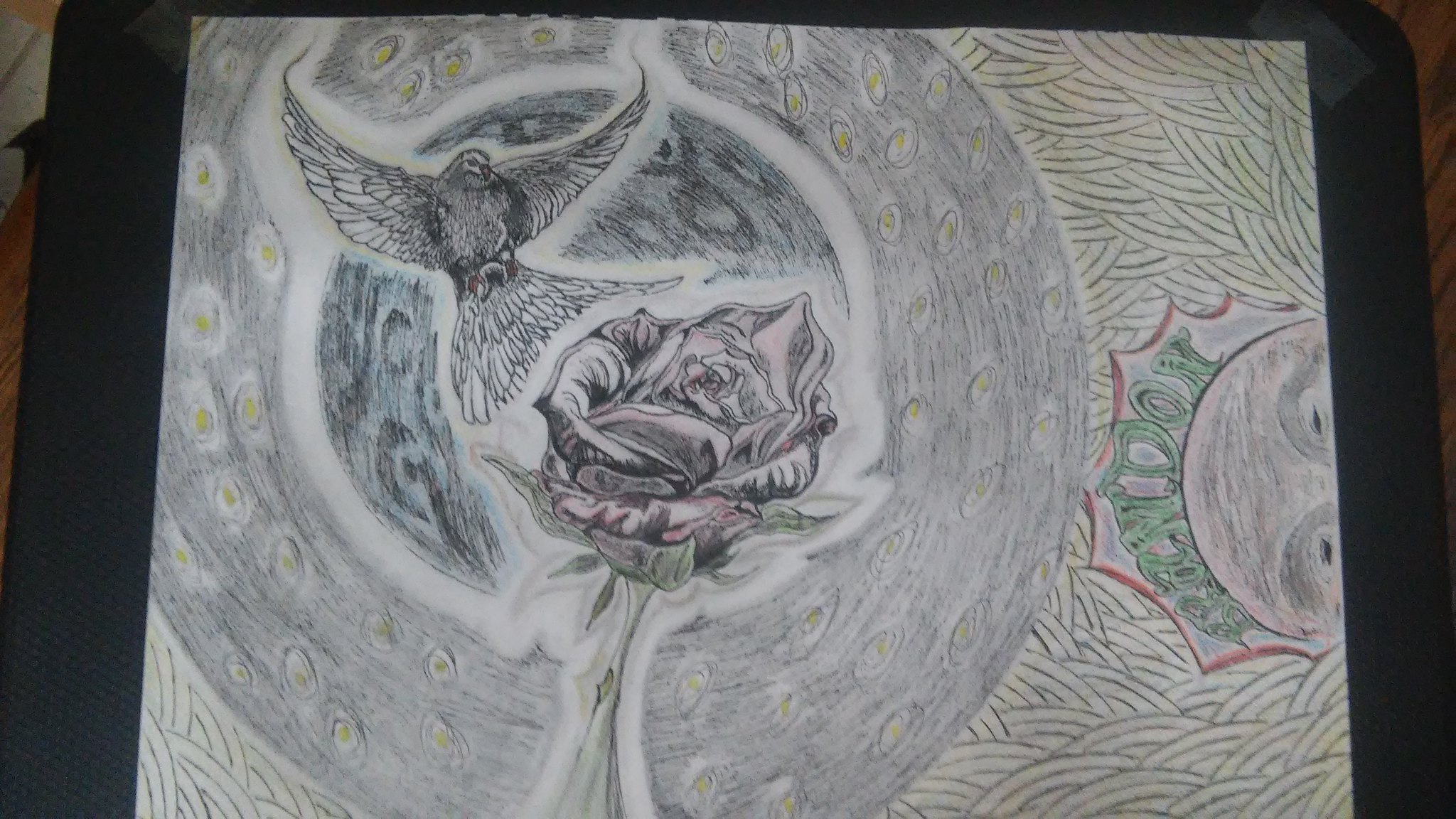This photograph captures a detailed and high-quality colored pencil drawing displayed on a tablet, situated on a black surface, possibly a table or a wall. The drawing features a beautifully rendered, black and white rose at its center. Above and to the left of the rose, a bird—likely a dove or an owl—is depicted with its wings fully spread as if about to land on the flower. The rose and bird are encircled by various design elements, including colored circles and a darker, almost moon-like circle, adding depth and complexity to the composition. On the left side, there is a black ring dotted with yellow circles, while on the right, a partially visible face peeks into the frame, distinguished by its eyes and subtle green writing above it. The picture's frame is black, with the entire scene set against what seems to be a wooden tabletop, providing a textured background for the detailed artwork.